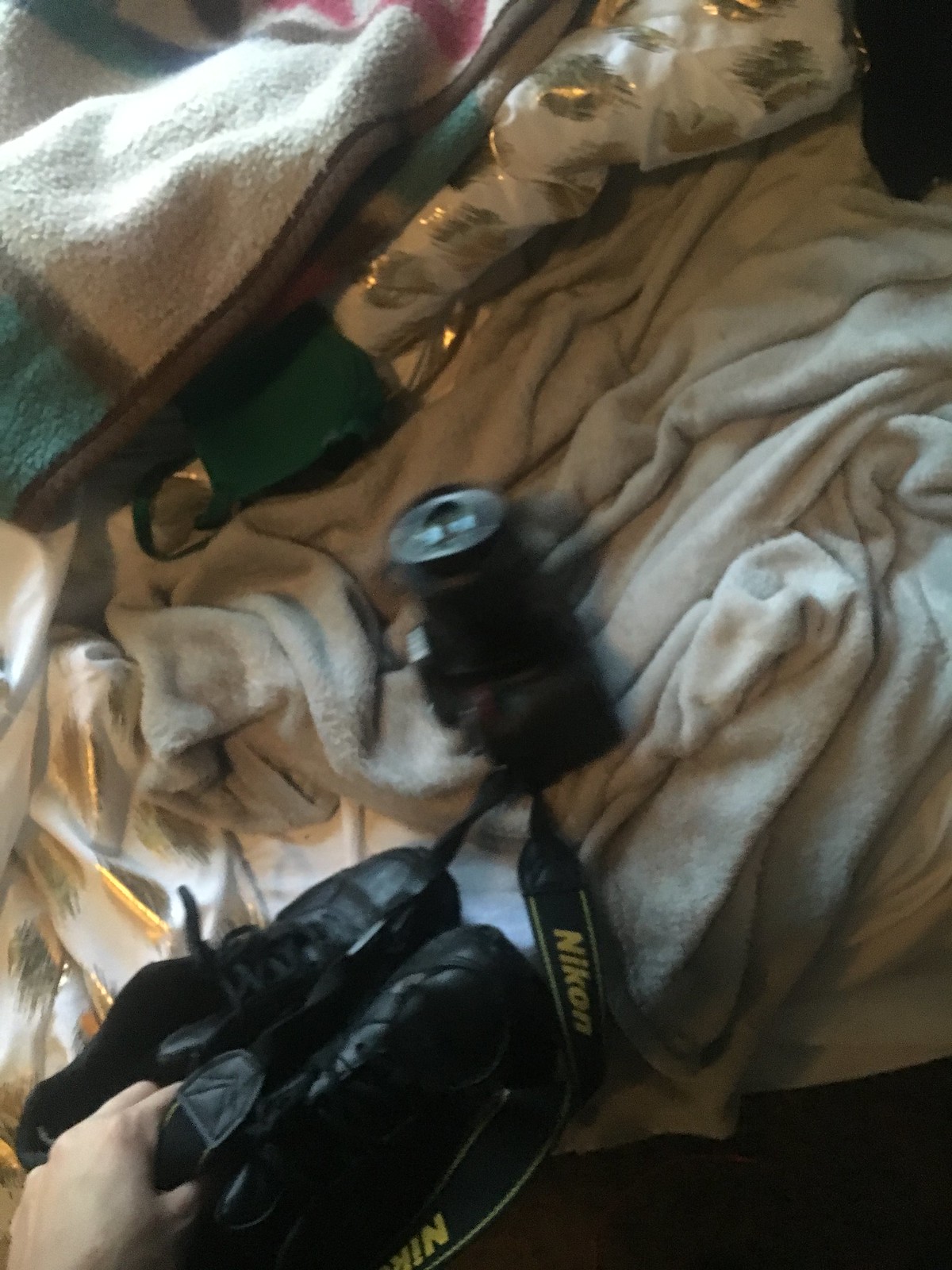A chaotic bedroom scene is depicted in this image. The bed is covered with rumpled silver and white sheets, with a disheveled gray blanket tossed casually at the foot. At the top of the bed, another blanket is visible among a collection of miscellaneous items in green and silver, whose exact nature is unclear. The focal point of the image is a slightly out-of-focus camera adorned with a recognizable Nikon strap, suggesting it has been hastily placed there. In the bottom left corner, a hand is captured mid-action, holding a pair of tennis shoes poised to be set down on the bed, likely next to the camera. The overall impression is that someone is in the midst of packing for a trip, with various personal belongings scattered across the unmade bed.